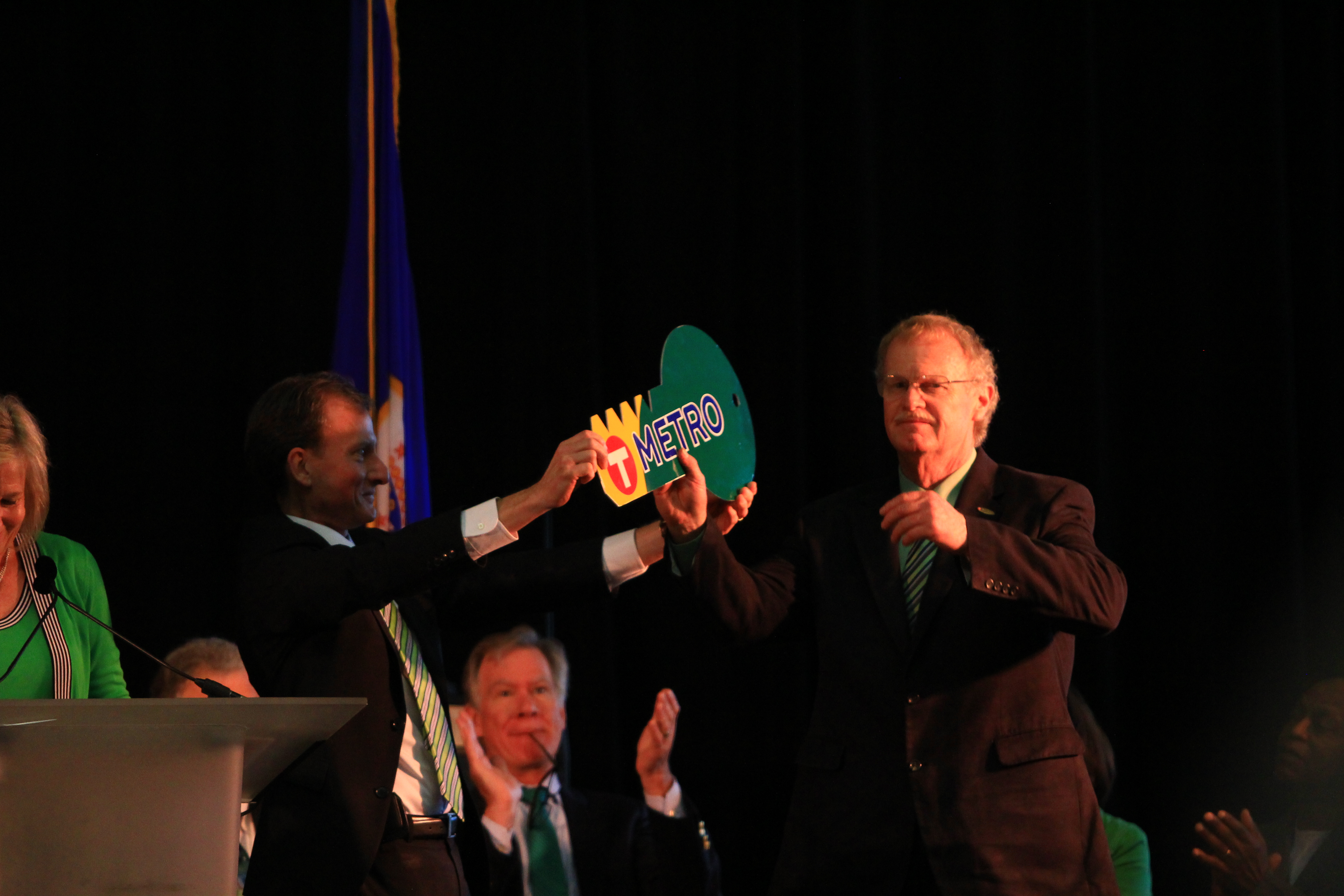In this image, we see a formal gathering, likely involving politicians or public officials. At the center of the scene, an older gentleman in a black suit, white undershirt, and striped tie—balding and wearing glasses—stands prominently. He reaches out with his right arm to receive a large, symbolic cardboard cutout of a key labeled "T Metro." The key, vividly colored in yellow and green with a white "T" inside an orange circle and the word "Metro" in blue with a white outline, is being handed to him by a slightly younger man also dressed formally in a black suit with a striped tie. 

To the left of this exchange, a woman in a green dress stands at a podium equipped with two microphones, appearing to make a speech. Her face is mostly obscured, but she is smiling, indicating her engagement in the event. In the background, which is somewhat dark and blurry, other participants are visible. An older man, possibly in his 50s or 60s, sits clapping with what might be a pen in his mouth, while another man in the bottom right corner is also seen clapping. The overall scene is staged with the focus on the presentation of the "T Metro" key, illuminated by artificial lighting, signifying an important ceremonial moment.